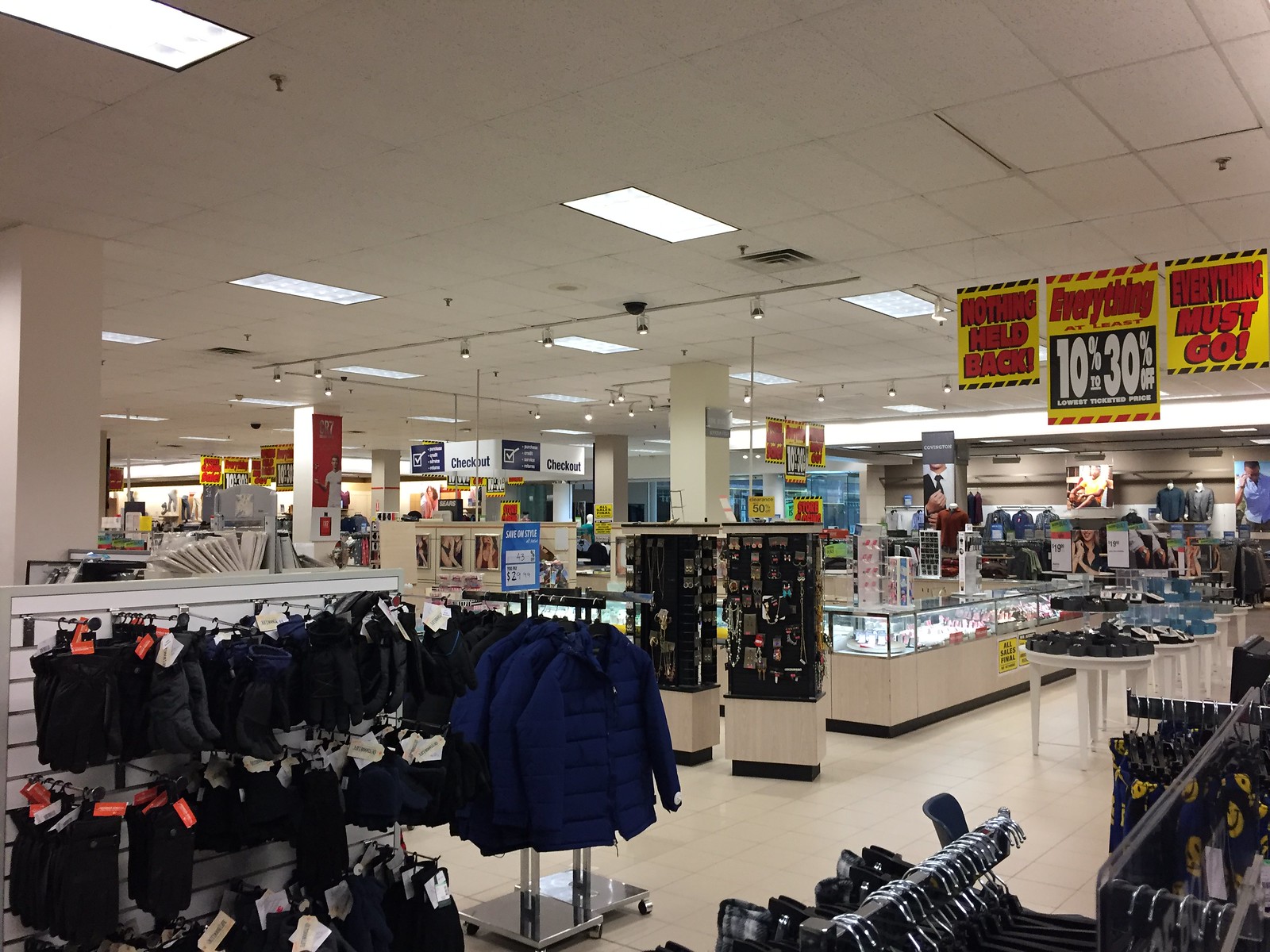This photograph captures the interior of a retail store currently hosting a clearance sale. A prominent sign hangs from the ceiling, featuring bold red text that reads, "Nothing Held Back, Everything Must Go," against a black backdrop with white lettering indicating discounts of "10 to 30% Off." 

In the foreground, a collection of thick navy winter jackets is showcased, with adjacent displays of black and gray gloves. Nearby, clothing racks present a variety of items, including a distinctive blue garment adorned with yellow smiley faces. 

Opposite the jackets, several jewelry displays are visible, showcasing necklaces and what appear to be earrings. Directly behind these displays, a larger glass jewelry counter can be seen. Overhead, fluorescent lights illuminate the store, which features a typical drop ceiling.